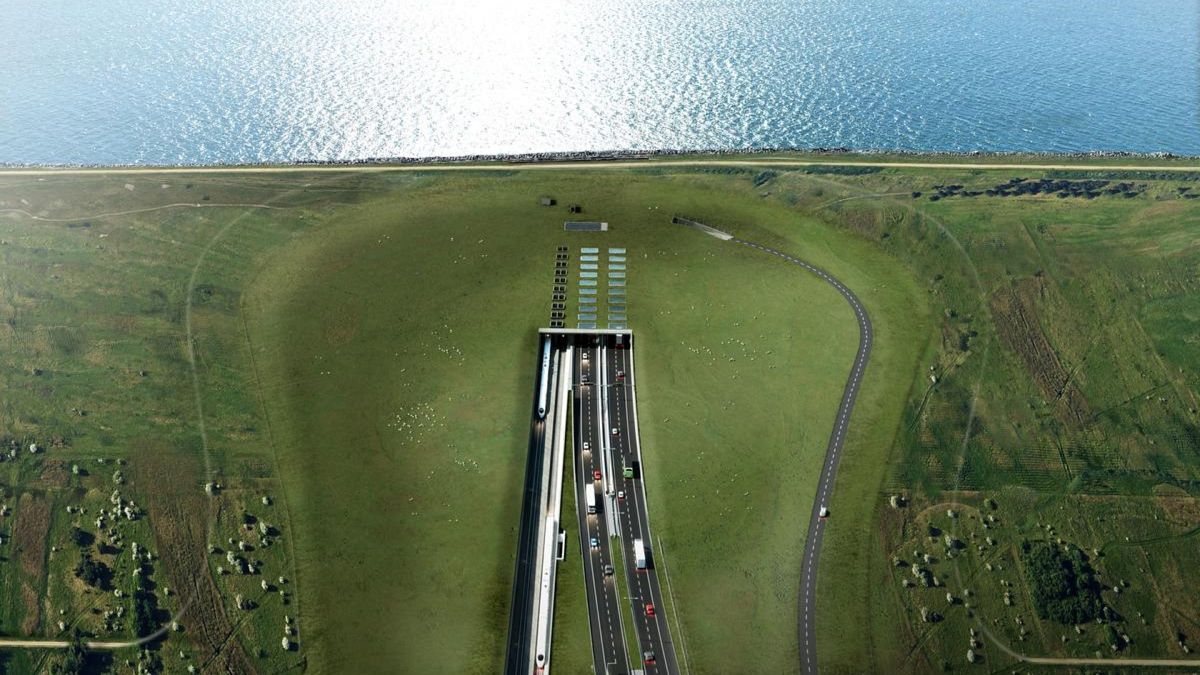The image showcases a detailed top-down illustration of a modern architectural setting featuring city traffic. At the top, a blue water body, possibly a sea or lake, glistens with a beam of light at its center, distinctly partitioned from the green land below. The land is predominantly covered in grassy fields with occasional trees, creating a scenery reminiscent of a golf course. The highway at the center of the image curves and descends into a tunnel that extends underneath the water body. Various miniature vehicles—cars, trucks, and a noticeable bullet train—navigate this road, emphasizing the bustling nature of the scene. The composition is well-balanced, with the lower half dominated by the greenery and the highway, while the upper half is characterized by the serene, reflective surface of the water.